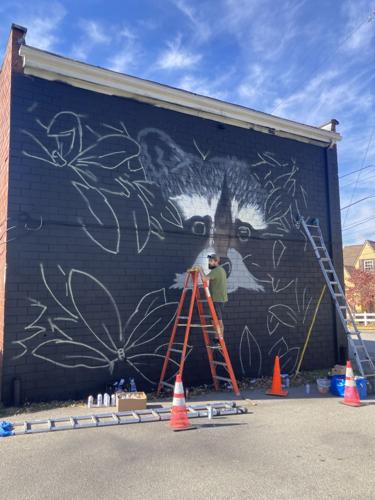The photograph captures a vibrant mural in progress on the angled side of a building, taken from a ground-level perspective under a bright blue sky with a smattering of white clouds. The mural center stage features an intricately detailed raccoon's face with gray, white, and brown markings, complemented by black eyes and nose. Surrounding the raccoon, the artist has outlined several flowers located towards the top left, top right, bottom left, and bottom right of the mural area. The man painting the mural is atop an orange ladder, dressed in a green shirt, hat, and shorts, and can be identified as a white man with a black beard. Below him, several cans of spray paint and a brown box rest on the light gray concrete, along with a flattened silver ladder and multiple safety cones—some solid orange, while others are orange and white striped. Further back, a tall silver ladder leans against the building. The mural itself stands out against a black background on the wall, creating a striking contrast with the splashes of color and intricate design elements of the artwork in progress.